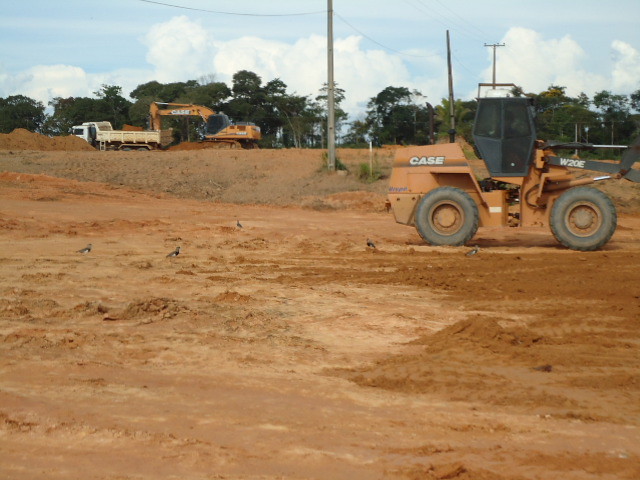This image captures an early-stage construction site set in a previously undeveloped field. The scene is bustling with activity, dominated by large construction vehicles emblazoned with the name "Case." Highlighted prominently is a Case W20E end loader with a black-painted cabin and oversized wheels, painted in a striking orange. This vehicle is actively unloading dirt into the back of an orange dump truck in the background. The ground is rough and uneven, indicative of the initial phases of land preparation—dirt and weeds are scattered about, suggesting a long way to go before any foundations can be laid. The site is punctuated by power poles and telephone lines, hinting at a nearby road. Surrounding the construction area are trees beneath a partly cloudy blue sky. The colors in the image are mostly earth tones—browns and oranges—accented by the blue sky, white clouds, and black elements of the machines. This detailed snapshot showcases a moment of transformation, as the machinery diligently works to reshape the landscape.